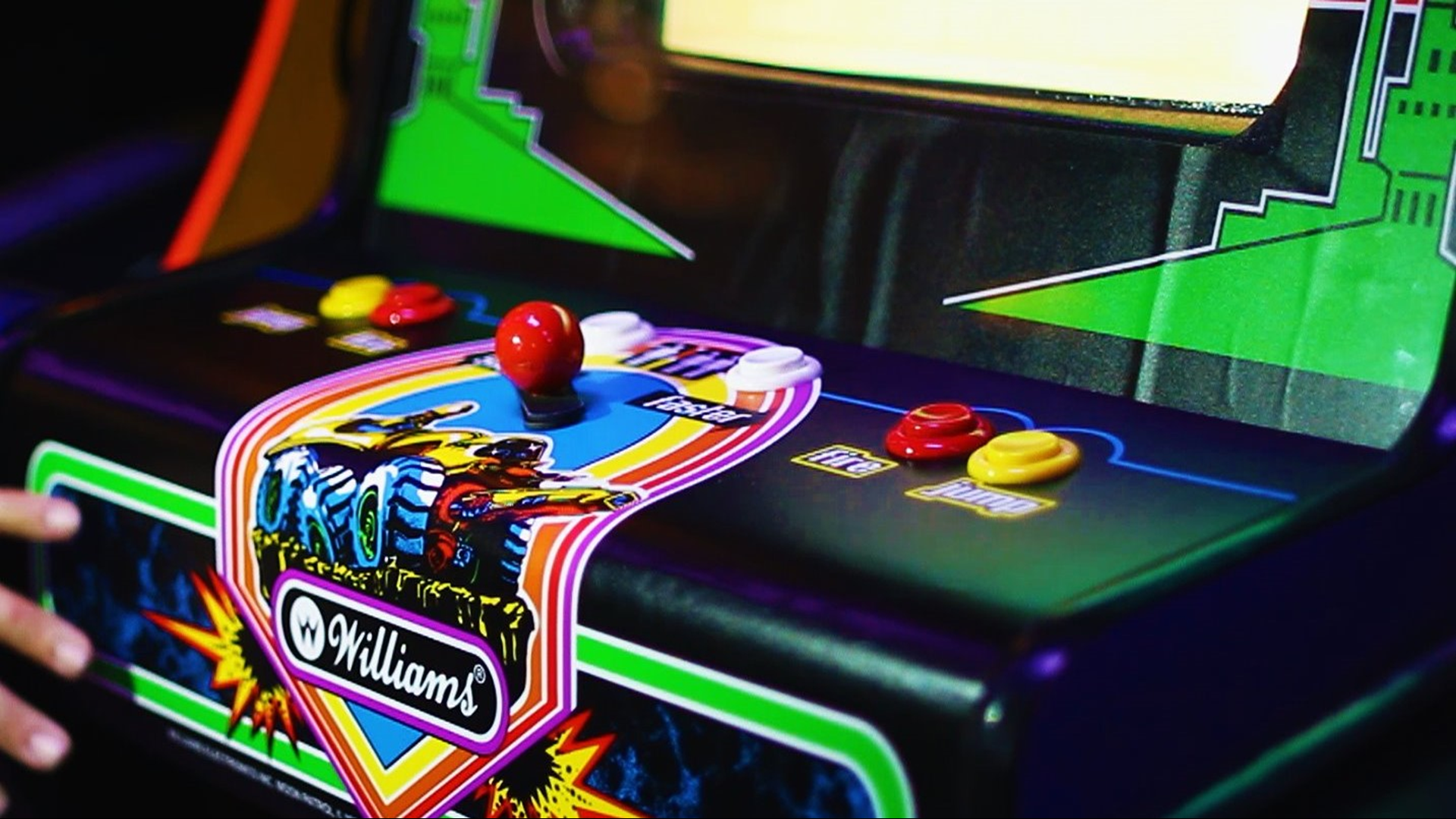The image is a close-up photograph focusing on the control panel of an old black arcade game machine, likely manufactured by Williams. Central to the panel is a red joystick encircled by a purple-bordered design with an additional triangular bottom. Two distinct buttons are positioned symmetrically on each side of the joystick—one red and one yellow on the left, and another set of red and yellow on the right. Above the joystick, two white buttons are noticeable. Lime green stickers accentuate various parts of the machine. The partial image includes an illustration of a brightly colored monster truck with explosive elements at the bottom of the visible area, and three fingers from an unseen person are visible at the lower left corner of the frame.